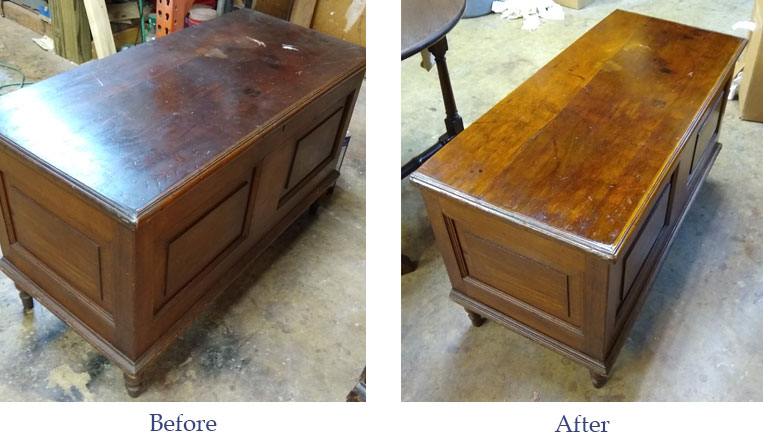This image consists of two side-by-side, before-and-after photographs of a wooden piece of furniture, possibly a chest, coffee table, or credenza, situated in a garage or workshop with a concrete floor. The left picture, labeled "before" in blue letters, shows a dark brown wooden piece with a lock on the front and significant wear on the top, including scratches, scuffs, and what seems to be white paint. Various objects are visible in the background. The right picture, labeled "after" in blue letters, depicts the same piece but lighter in color, shinier, and less worn, indicating it has been sanded and re-varnished. Although some scuffs remain, they are significantly buffed out. Both images reveal additional furniture in the background, such as another table in the upper left-hand corner, emphasizing the workshop setting.